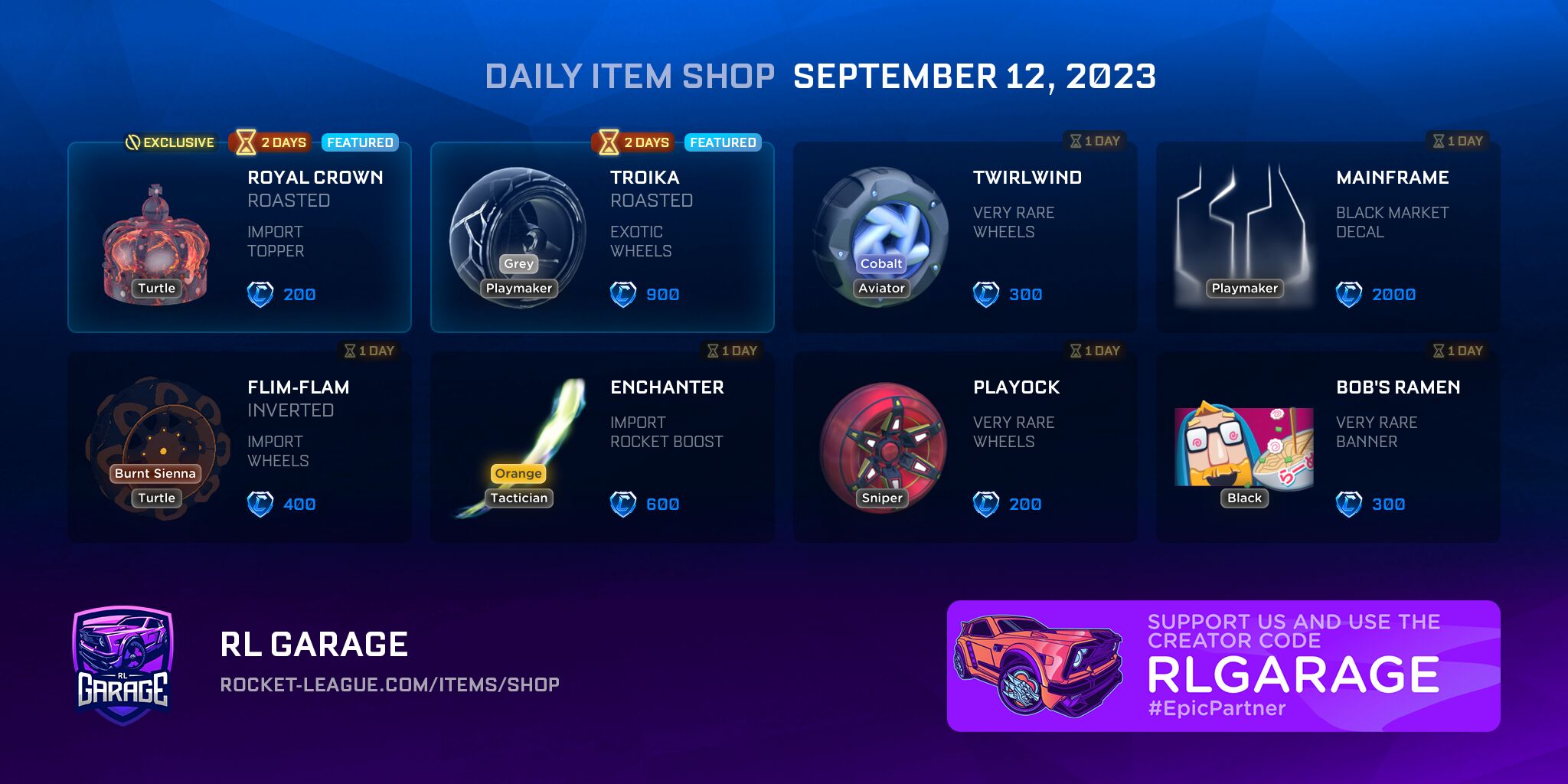This is a screenshot of a "Rocket League" video game's daily item shop, captured on September 12, 2023. The image is landscape in orientation, featuring a background that transitions from blue at the top to dark blue-purple at the bottom. 

At the top center, the text "Daily Item Shop" is displayed in grey letters, while the date is shown in white letters beneath it. The shop is organized into two rows, each containing four items available for purchase.

In the first row, the items listed are:
1. **Exclusive Royal Crown Roasted**
2. **Troika** - This item is labeled with "Two days remaining" and marked as "Featured," and it resembles some type of wheel.
3. **Twirl Wind**
4. **Mainframe**

In the second row, the items available are:
1. **Flim Flam**
2. **Enchanter**
3. **Playak**
4. **Bob's Ramen** 

These items appear to be various upgrades or customizations available for purchase within the game.

At the bottom left corner of the screenshot, there is an icon of a shield with a truck on it, labeled "Garage." To the right of this icon, the text "RL Garage rocket-league.com/items/shop" is displayed in white letters. Additionally, it prompts players to "Support us and use creator code RL Garage."

This image illustrates the in-game item shop where players can buy add-ons for the game "Rocket League."